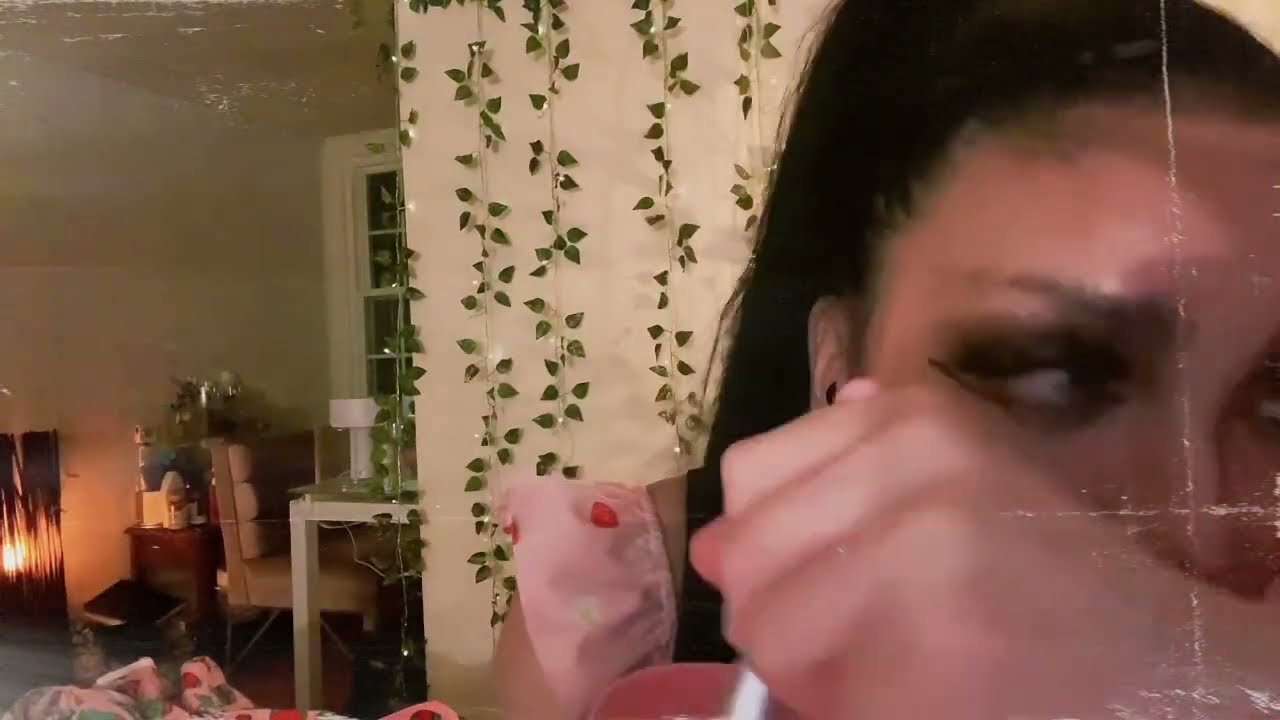The image captures a close-up of a woman, likely presenting as Latino, in a residential setting. She is positioned on the right side and appears to be in motion, potentially sneezing into her left wrist. Her face is partially obscured by her left fist, held in front of her mouth, while her eyes are closed. She has noticeable dark makeup with winged eyeliner and heavy eyelash makeup. The woman is wearing a pink dress with a noticeable puffed sleeve on her right shoulder. Her dark hair is pulled back tightly into a ponytail. In the background to the left, there is a wall adorned with decorative fake greenery vines and possibly Christmas lights. Further left, the room opens up into a cluttered living room area featuring a white curtain with a green leaf pattern, a fireplace, a table with a window above it, and a chair that resembles a kitchen chair but with upholstery. There's also a nightstand cluttered with bottles or containers, and in the lower left corner, there appears to be a black wastepaper basket, possibly with a blanket in the foreground.